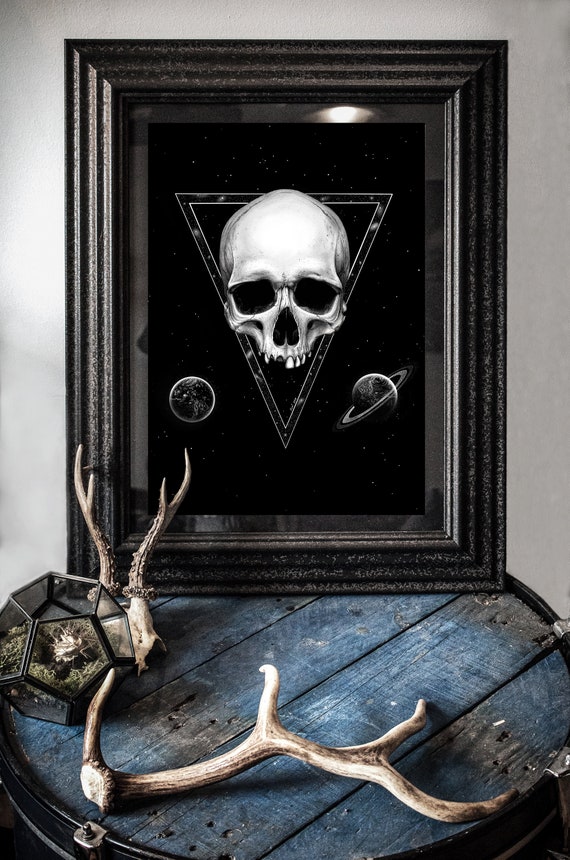A black-framed picture with a black mat and a light, starry background depicts two planets and the upper half of a skull within a white-bordered triangle. The skull, missing its lower jaw, creates a stark contrast against the dark backdrop. The image is accentuated by a starry night-like black background. The frame rests on a blue, wooden barrel top. Nearby on the barrel, there are antlers and possibly a terrarium or geodesic holder, adding a unique touch to the scene. Bones, resembling a hand and another bone fragment, also lie on the barrel, enhancing the eerie ambiance of the setup.